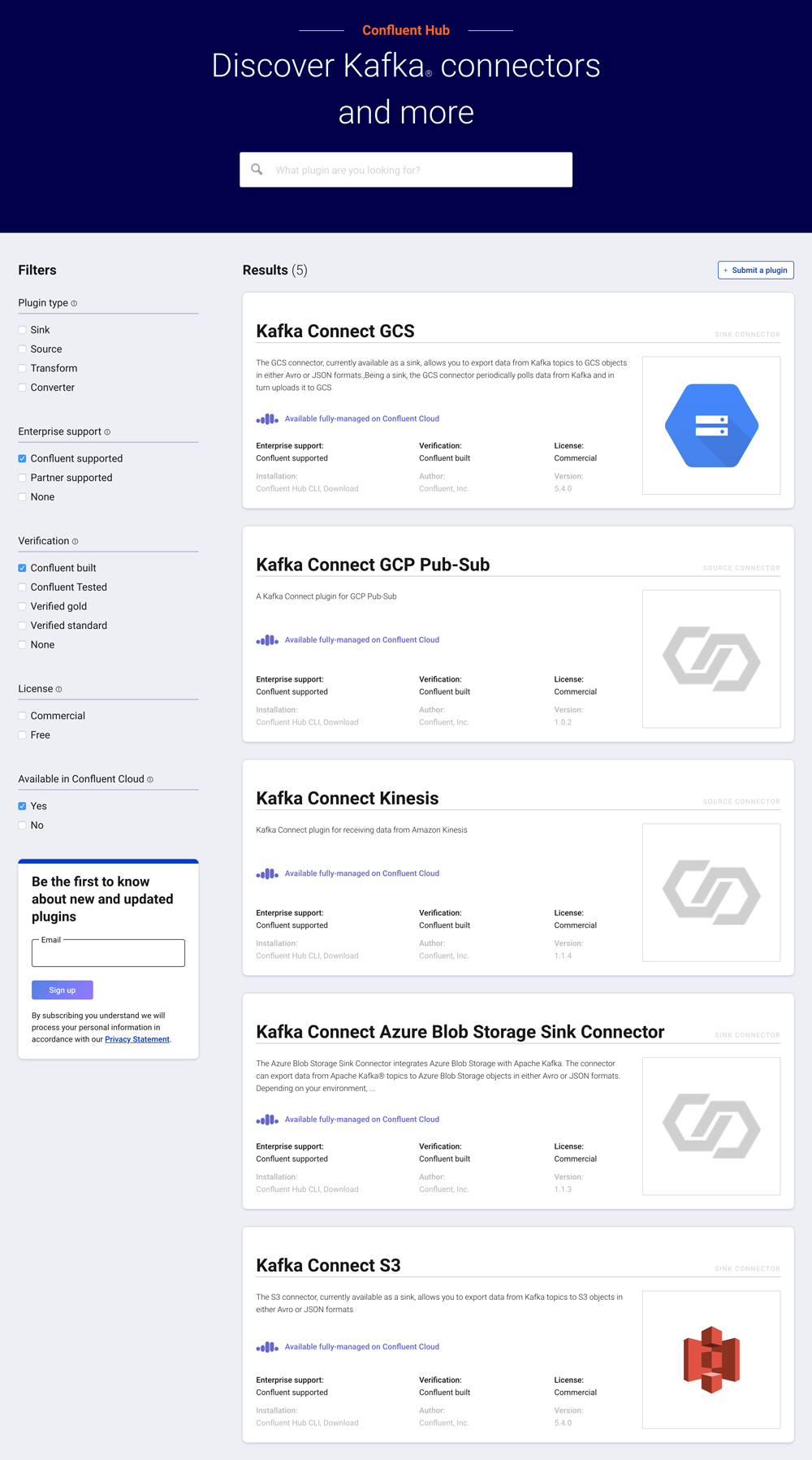This is a screenshot of the Confluent Hub website's front page, which is designed for discovering Kafka Connectors and more. At the top of the page, the heading "Confluent Hub" is prominently displayed, followed by the subtitle "Discover Kafka Connectors." Beneath this heading, there is a search bar for users to easily find specific connectors.

Under the search bar, there's a section labeled "Results" that showcases five Kafka Connectors:
1. Kafka Connect GCS
2. Kafka Connect GCP PubSub
3. Kafka Connect Kinesis
4. Kafka Connect Azure Blob Storage Sync Connector
5. Kafka Connect S3

Further down, various filters allow users to refine their search. The filters include:
- Plugin Type: Sync, Source, Transform, Converter
- Enterprise Support: Confluent Supported, Partner Supported, None
- Verification: Confluent Built, Confluent Tested, Verified Gold, Verified Standard, None
- License: Commercial or Free
- Availability in Confluent Cloud: Yes or No

Additional information includes a blurb encouraging users to subscribe for updates on new and updated plugins. Users can enter their email address and click "Sign Up," with a disclaimer that subscribing means their personal information will be processed according to the privacy statement.

At the top of the page, there is also a prominent white button with blue letters labeled "Submit a Plugin," allowing users to submit their own plugins for inclusion on the site.